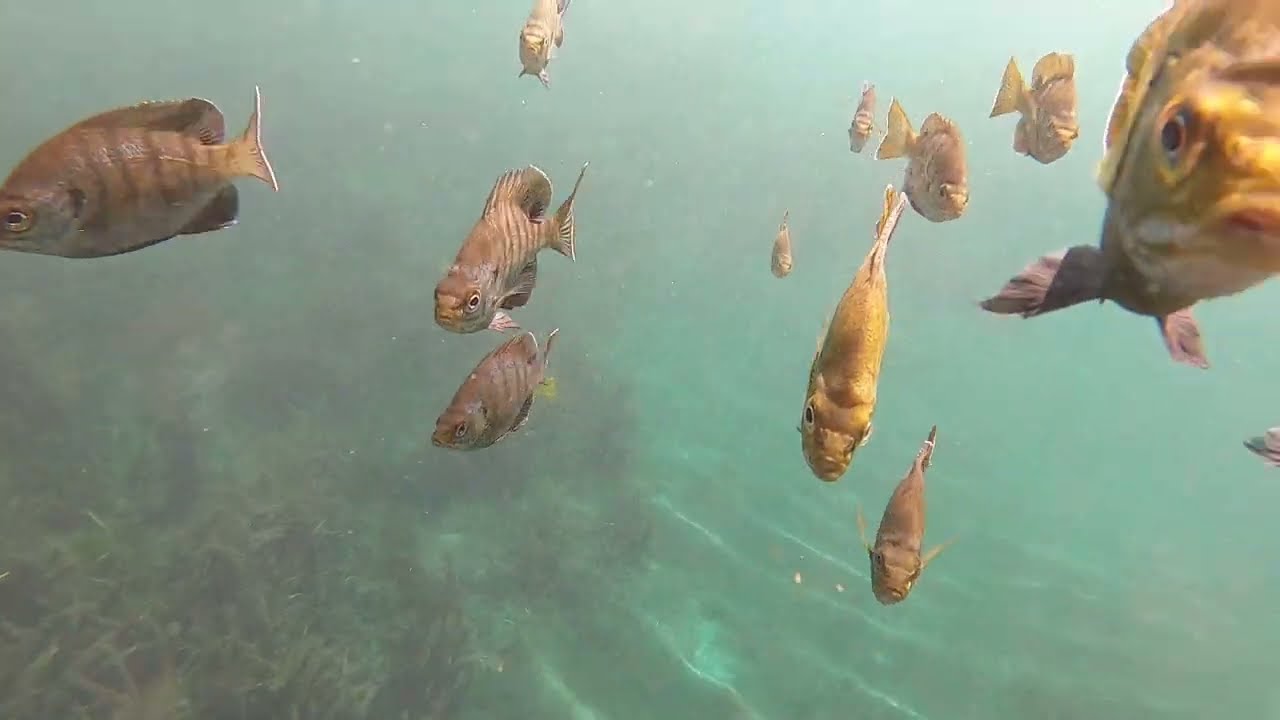In this underwater scene captured in the shallow, clear waters of Gambier, the image reveals a murky mix of greenish and bluish hues, illuminated by light refracted from the water’s surface. Dominating the scene is a school of approximately 10 to 12 fish, primarily featuring lightly striped patterns in shades of gold, brown, and yellow. These fish, similar in size and marked by around six stripes each, swim collectively towards the camera, with some appearing to dive beneath an unseen snorkeler. On the left side, a coral reef stands out, while the bottom right and the right side of the image display patches of vegetation. Additionally, a striped gray fish with a large dorsal fin can be seen along with a few yellowish fish, randomly dispersed, enhancing the scene's vibrant diversity. The overall backdrop of sand reflects intricate light patterns, contributing to the ethereal quality of this captivating underwater vista.